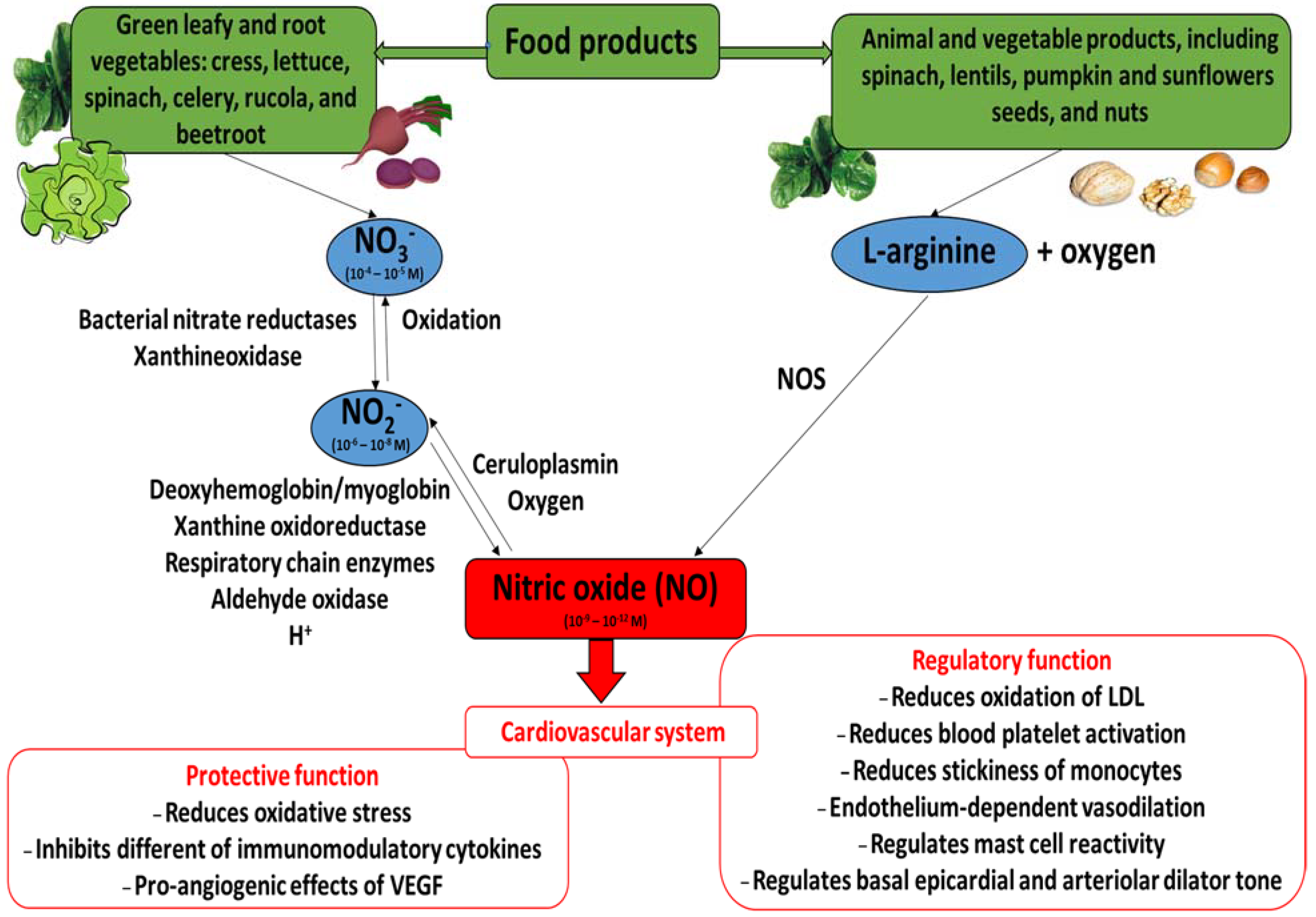This image is a detailed diagram illustrating the process of how the body utilizes certain plant and animal products to produce nitric oxide, contributing to cardiovascular health. At the top, there is a green box labeled "Green Leafy and Root Vegetables" listing cress, lettuce, spinach, celery, rucola, and beetroot. An arrow points from this box to another box labeled "Food Products." From the "Food Products" box, arrows extend left and right. 

To the left, the diagram details that these vegetables undergo bacterial nitrate reductases and various oxidative processes to produce nitric oxide (NO), marked in a red box at the bottom. This NO is shown to have several cardiovascular protective functions, including reducing oxidative stress, inhibiting immunomodulatory cytokines, and facilitating pro-angiogenic effects of VEGF.

To the right, a green box lists "Animal and Vegetable Products," including spinach, lentils, pumpkin, sunflower seeds, and nuts. This section highlights that these products produce L-arginine, which also leads to the production of nitric oxide. The nitric oxide from this pathway is involved in multiple cardiovascular functions such as regulating vascular tone, inhibiting blood platelet activation, and reducing LDL oxidation.

The entire diagram is set against a white background with lines and arrows connecting various components, breaking down the chemical processes and compounds involved.